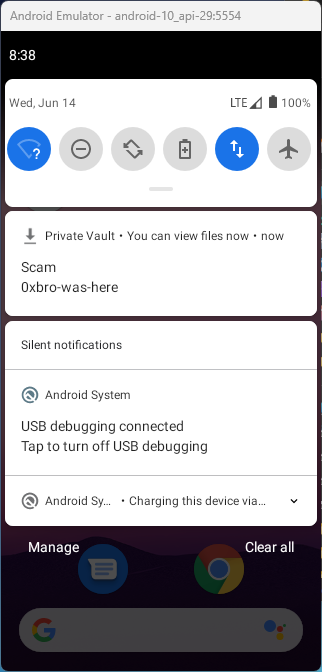The image is a screen capture taken from a mobile device, displaying three vertically stacked rectangular windows with curved corners, set against a black background. The top of the screen features a white bar with gray text that reads "Android Emulator - Android-10_API-29:5554," and to the left, the time is displayed as 8:38.

The first window, positioned directly beneath the time, is white and populated with several icons. Below this is the second white window, which contains several lines of text. At the top of this window, it reads, "Private Vault. You can view files now." The third and final window is also white and rests below the second. The top of this window contains the prompt "Silence Notifications."

Overall, the image is a detailed screen capture showcasing the layered interface of an Android emulator, with distinct sections dedicated to icons, file viewing options, and notification settings.